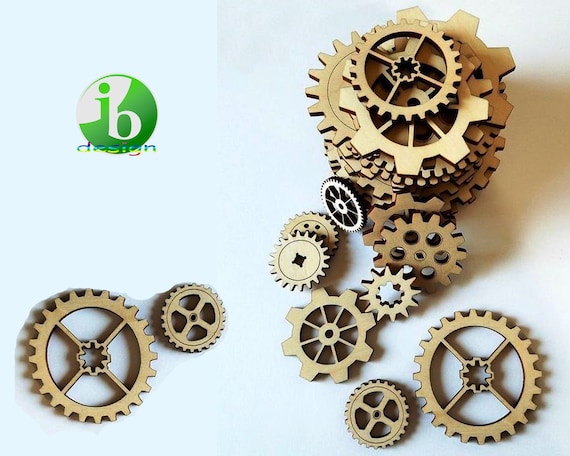The image prominently features a variety of gears scattered across a light background. In the bottom left corner, there are two light brown gears lying flat. The top right portion of the image showcases a pile of gears of different sizes and shapes, with larger ones at the base and smaller ones on top. Some gears are leaning against the pile, while others are strewn about towards the bottom right corner. The background appears to be a mix of blue and white tones, adding a contrast that emphasizes the gears. 

A logo is visible in the image, reading "I, Bee Design." The logo features alternating white and green colors, where the "I" is green and the "Bee" is white, set against opposite colored backgrounds. The details of the logo are somewhat pixelated, making it blend slightly into the surrounding scene.

Overall, the image integrates a design theme with an array of intricately arranged gears, creating a complex and visually engaging composition.